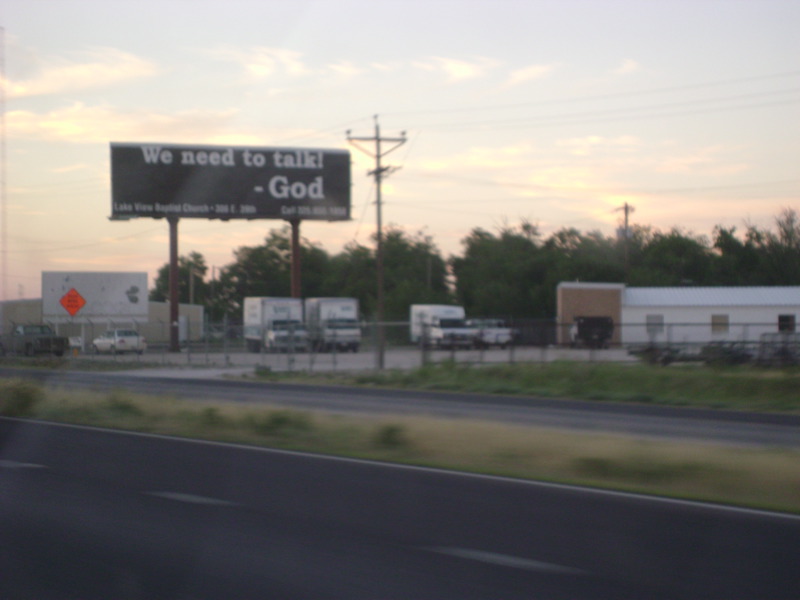The photograph captures a serene outdoor scene taken in the late evening, just as the Sun is setting or has recently set. The sky transitions beautifully from a very light gray-blue near the top to a soft pink closer to the horizon, creating a gradient that vividly showcases the day's end. Bright yellow hues illuminate the scattered clouds, adding warmth and depth to the image.

In the foreground, a roadway, possibly a highway, stretches out with clearly marked white dashed lines. This road is flanked by a strip of vibrant green grass, adding a touch of nature to the otherwise built environment. Beyond the grass, there stands a commercial building, indicative of an industrial area. Several white shipping-style trucks are parked in an orderly fashion within the adjacent parking lot, suggesting the location is a hub of activity during business hours.

Prominently, a large black sign with crisp white font catches the eye. It reads, "We need to talk - God." This intriguing message adds a thought-provoking element to the tranquil evening scene, inviting viewers to reflect amidst the picturesque backdrop.